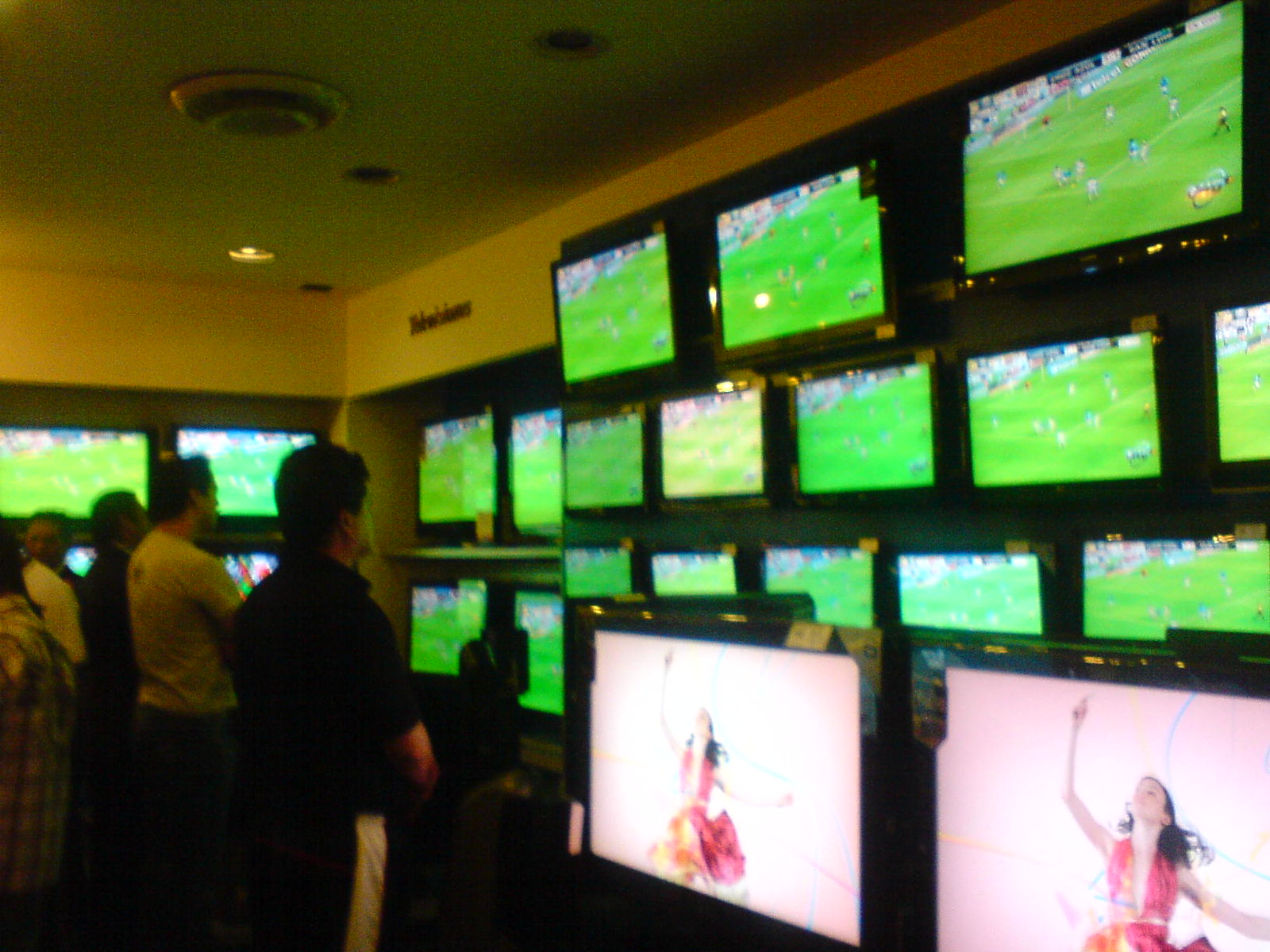The image captures a somewhat grainy, yet detailed scene inside an electronics store featuring a tremendous wall of modern flat-screen TVs. The majority of these televisions display a vivid greenish scene of a soccer game, covering rows from the ceiling down to waist height. In the bottom right corner of the wall, two larger screens diverge from the soccer broadcast, instead showing a woman in a red and orange dress dancing against a white backdrop. A white ceiling with recessed lighting and a circular vent is visible above the wall of TVs, along with the word "TELEVISIONS" written in bold black letters. Five casually dressed men—sporting a mix of athletic and street clothes—stand in front of the screens. Two of these men have their arms crossed, while others engage with each other, all engrossed by the vibrant displays.